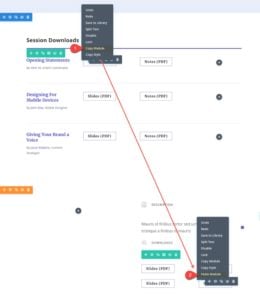This is a low-quality, small, and blurry screenshot. Despite its obscurity, a few elements can be identified. At the very top, there's a light blue bar, which is notably empty. Just below, situated in the upper left corner, is a small blue rectangle featuring illegible white text, possibly the website's logo. 

Directly underneath this area, there is text that reads "session downloads" in a clear black font—the only readable content on the page. Adjacent to this text is an open dropdown menu in dark charcoal gray, showcasing several entries in white font. 

Further down the page, there are three distinct rectangles lined up vertically. Each rectangle contains an entry written in blue font, which remains unreadable, alongside two clickable buttons in white, with black text. At the end of each entry on the right-hand side, there are black circular buttons, all of which appear to have been clicked.

Below these elements lies an orange rectangle with white font, though the text is also indecipherable. Finally, at the bottom of the image, there is a second open dropdown menu, similarly colored in charcoal gray.